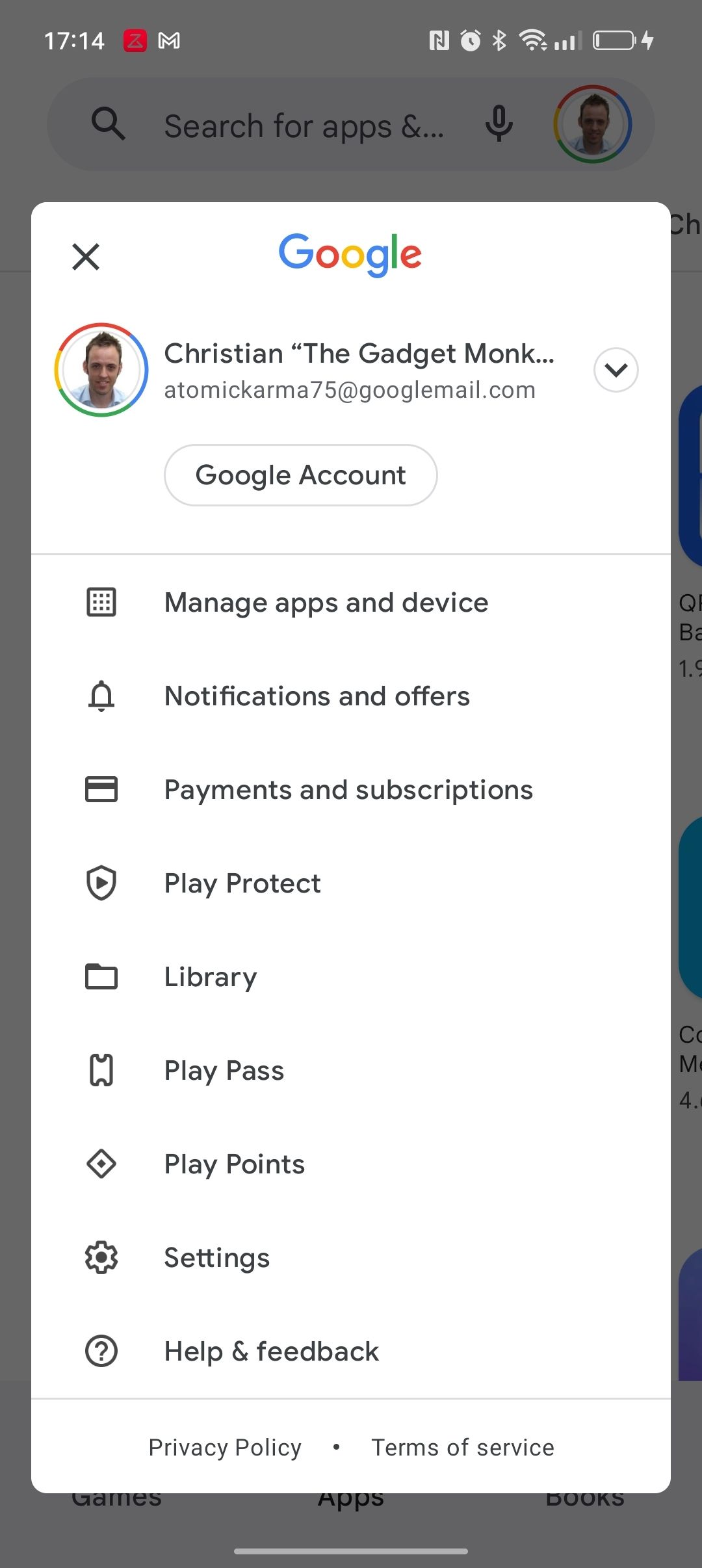This detailed caption provides an in-depth description of a screenshot taken from someone's phone showcasing their Google settings page:

---

The screenshot is captured from a smartphone displaying the Google settings interface. The background is slightly grayed out, and at the very top of the screen, the time is shown in 24-hour format as 17:14. Also visible at the top are standard status icons including an alarm, Bluetooth, Wi-Fi, signal strength, and a nearly depleted battery that is presently charging.

Directly below these icons is the Google search bar, accompanied by a small profile picture of the user. The main portion of the screen showcases the Google settings menu within a white box. At the apex of this box, the bold title "Google" is displayed, followed by the user’s name, “Christian the Gadget Monk,” alongside Christian's email address and the label "Google account."

Listed down the screen, various options are available: "Manage apps and device," "Notifications and offers," "Payments and subscriptions," "Play Protect," "Library," "Play Pass," "Play Points," "Settings," "Help," and "Feedback." At the very bottom of the menu are links to the "Privacy Policy" and "Terms of Service."

Christian's profile picture, set within the colorful Google circle at the top of the page, depicts a male with short hair styled slightly longer and standing up at the top. He is wearing a blue shirt.

---
This caption provides a comprehensive and visually descriptive narrative of the screenshot, detailing the interface elements and the visible user profile.